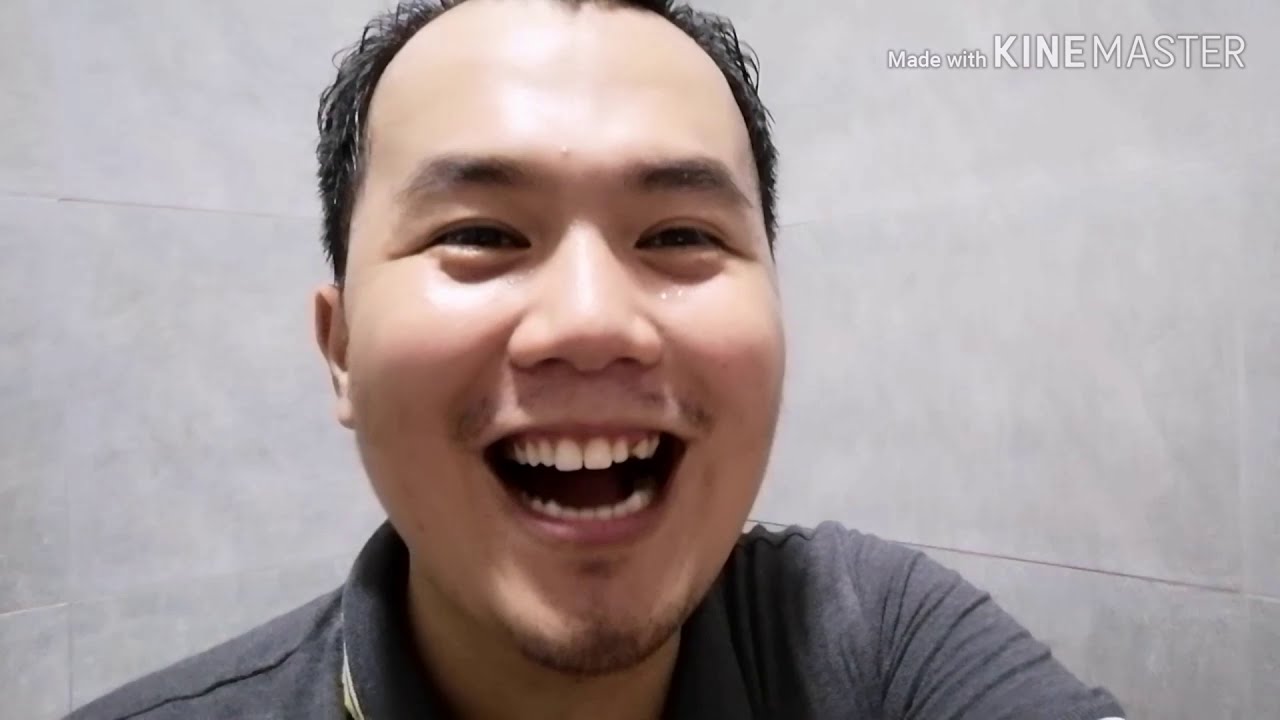In this photo, a smiling Asian man with light skin and short black hair is captured, seemingly taking a selfie. His expression is one of happiness and excitement, as evidenced by his wide smile with open mouth and smiling eyes. He has a faint goatee and a slight mustache. The man is wearing a gray collared polo shirt, and fine details like a line at the collar are visible. The background is a light gray wall with some linear patterns, suggesting it might be tiled, possibly indicating a bathroom or shower stall setting. In the upper right corner of the image, the text "MADE WITH KineMaster" is prominently displayed, with "Kine" being bolded. The overall scene is very focused on the man, who is central and very close to the camera.